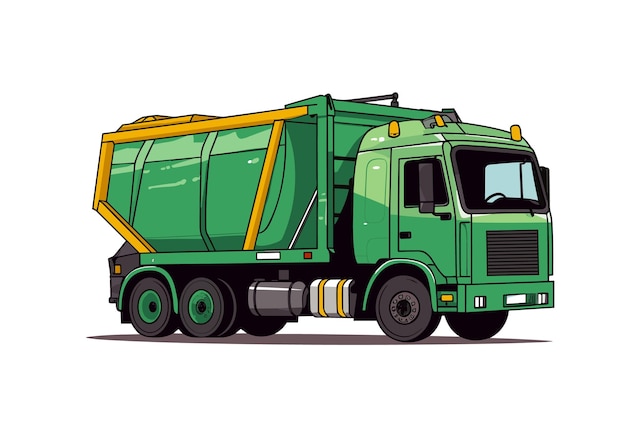The image depicts a detailed, cartoon-like drawing of a green garbage truck with light green highlights. The truck is outlined with a white border and positioned on a gray area, likely representing a street. Emphasizing its functionality and design, the truck is adorned with yellow railings and orange structural girders around its body, suggesting support beams. The truck's cab features a prominent black grille, and through the blue-tinted windshield and driver's side window, the truck's interior is partially visible. The truck heads towards the right side of the image, casting a shadow beneath it.

On the passenger side, three tires are visible, including a set of rear dually wheels with green centers to match the truck’s body color. Additional details include three orange cab lights on top and a silver rectangle with two vertical gold bands behind the passenger door. The truck's back fender is also green, and there is a noticeable silver area with yellow stripes, possibly representing a fuel tank or storage compartment, adding further intricacy to this high-quality digital drawing.